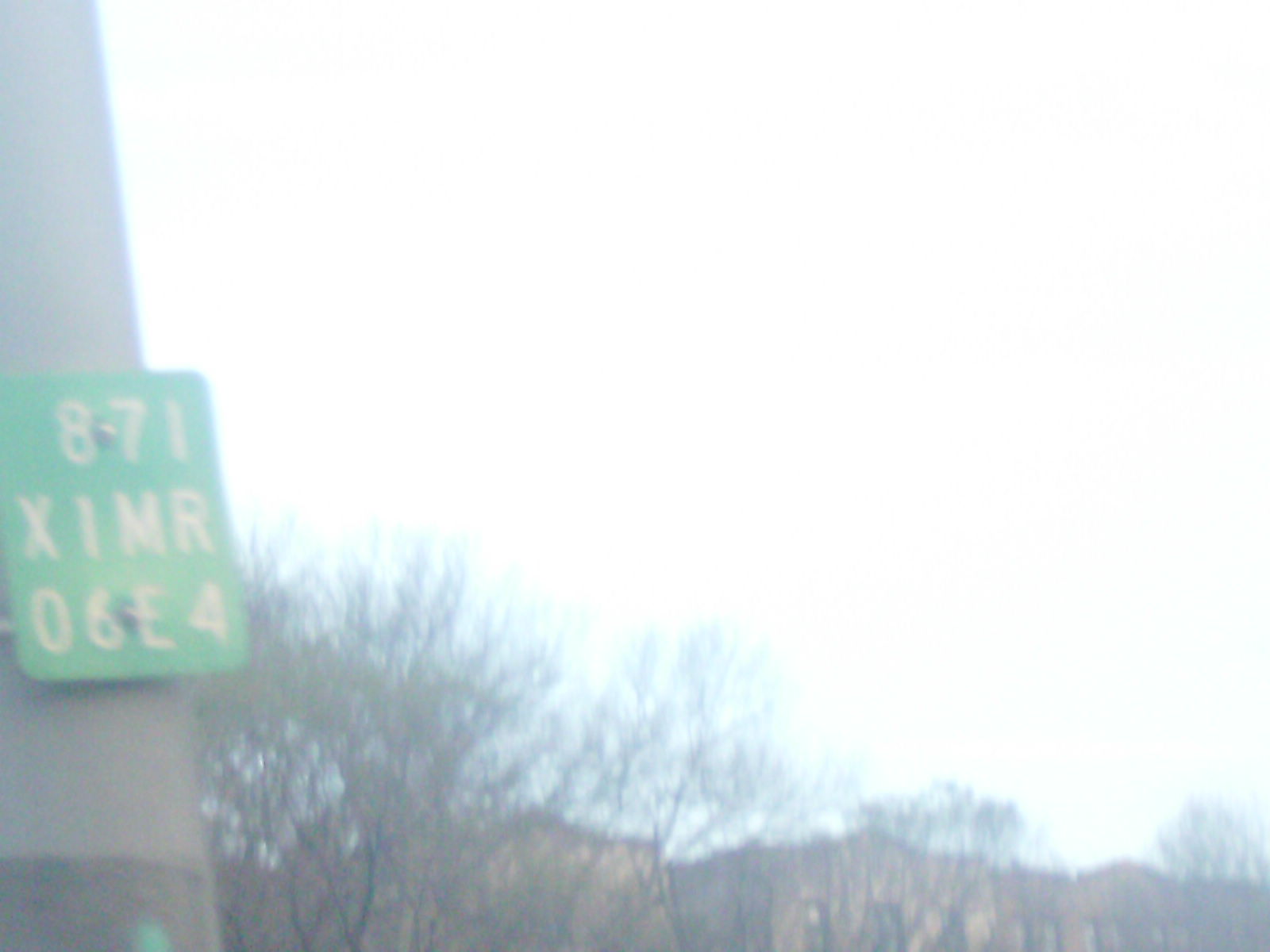This blurred, washed-out digital color photo captures an outdoor scene under a bright, clear sky, though the sky appears washed out at the top right. The image shows barren trees and rolling hills in the distant background. Dominating the left side of the picture is a large concrete pole, extending from the top left to the bottom left, supporting a green street sign with white lettering that reads "871-XIMR-06E4." Despite some hints of potential background structures, like buildings, the overall scene is predominantly defined by the overwhelming brightness and blurry focus, giving it a somewhat unclear and indistinct appearance.